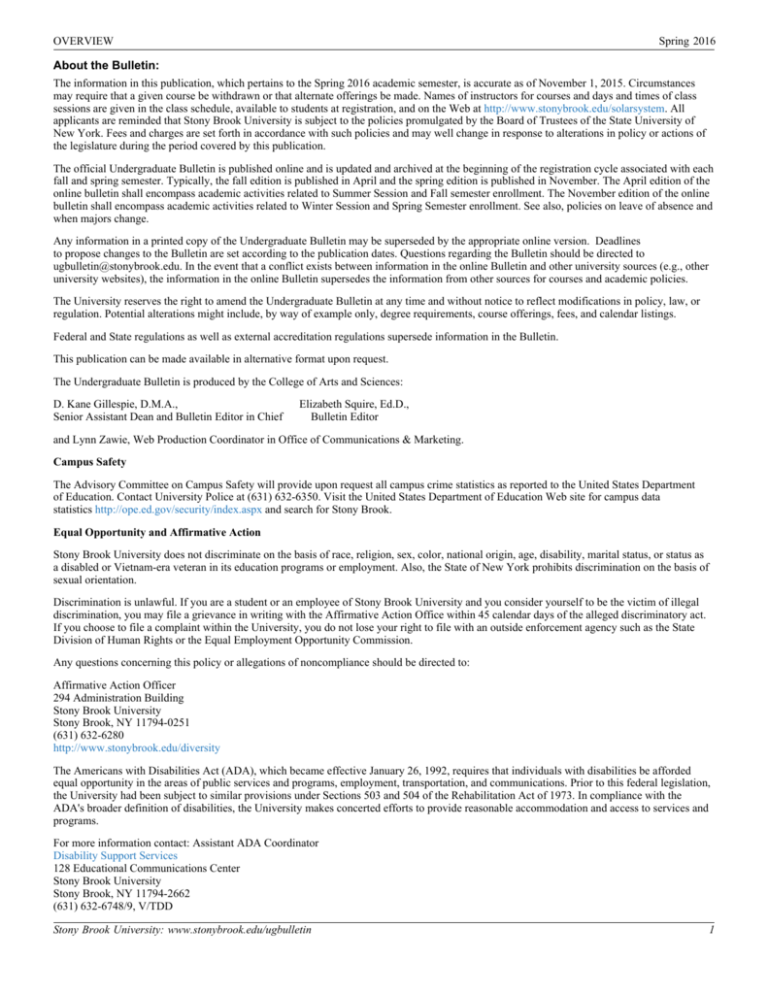Here's a detailed, cleaned-up caption for the image:

---

The image is a vertically-oriented rectangular document, depicting an official bulletin from Stony Brook University. At the very top of the document, there is a header with the word "Overview" aligned to the left, and "Spring 2016" aligned to the right. A thin line runs underneath this header, demarcating it from the main content below. 

Immediately following the line, the main body of the document starts with the heading "About the Bulletin." The text informs the reader that the information presented pertains to the Spring 2016 academic semester and is accurate as of November 1st, 2015. It includes a disclaimer that courses listed may be withdrawn and substituted with alternative offerings. Additionally, details such as course instructors, schedules, and session timings are provided in the class schedule, accessible to students during registration and online at www.stonybrook.edu/solarsystems.

At the bottom, another thin line separates the main content from the footer, where "Stony Brook University" is prominently displayed. The bulletin concludes by reminding applicants that the University adheres to policies set by the Board of Trustees of the State University of New York. It also notes that fees and charges are determined in accordance with these policies and may be subject to change based on new legislative actions during the publication period.

---